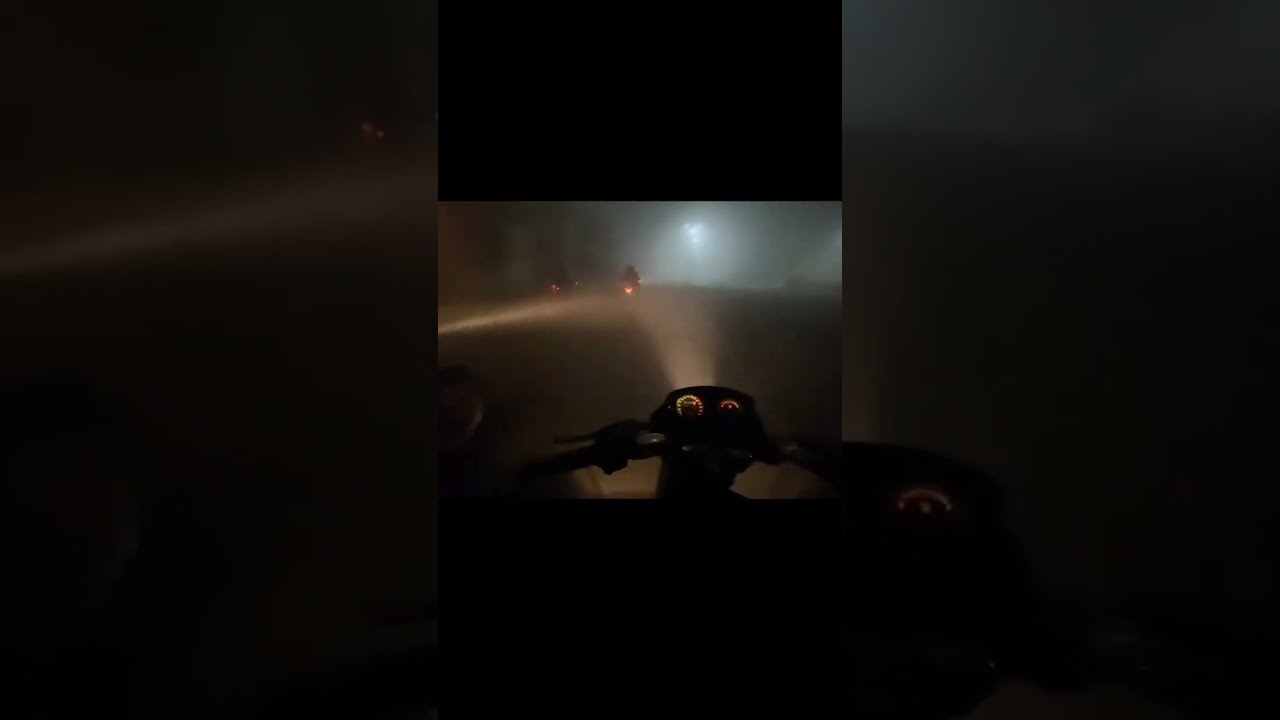This image depicts a nighttime scene captured from the perspective of a rider on a motorcycle, possibly with a helmet-mounted camera. The vertically rectangular picture features a central, colored photograph displaying the illuminated gauges and handlebars of the motorcycle, from which a headlight beams forward, illuminating the road ahead. The scene is enveloped in fog, adding to the overall darkness and creating a hazy, mysterious atmosphere. Ahead of the rider, a couple of motorcycles, identifiable by their tail lights, are visible against the otherwise empty road. In the distance, a large street lamp punctuates the obscurity, casting a faint glow in the murky surroundings. The surrounding background consists of a darkened, blurred close-up of the central image, which adds to the sense of motion and depth, emphasizing the solitary, nocturnal journey through what appears to be a rural or less densely populated area.